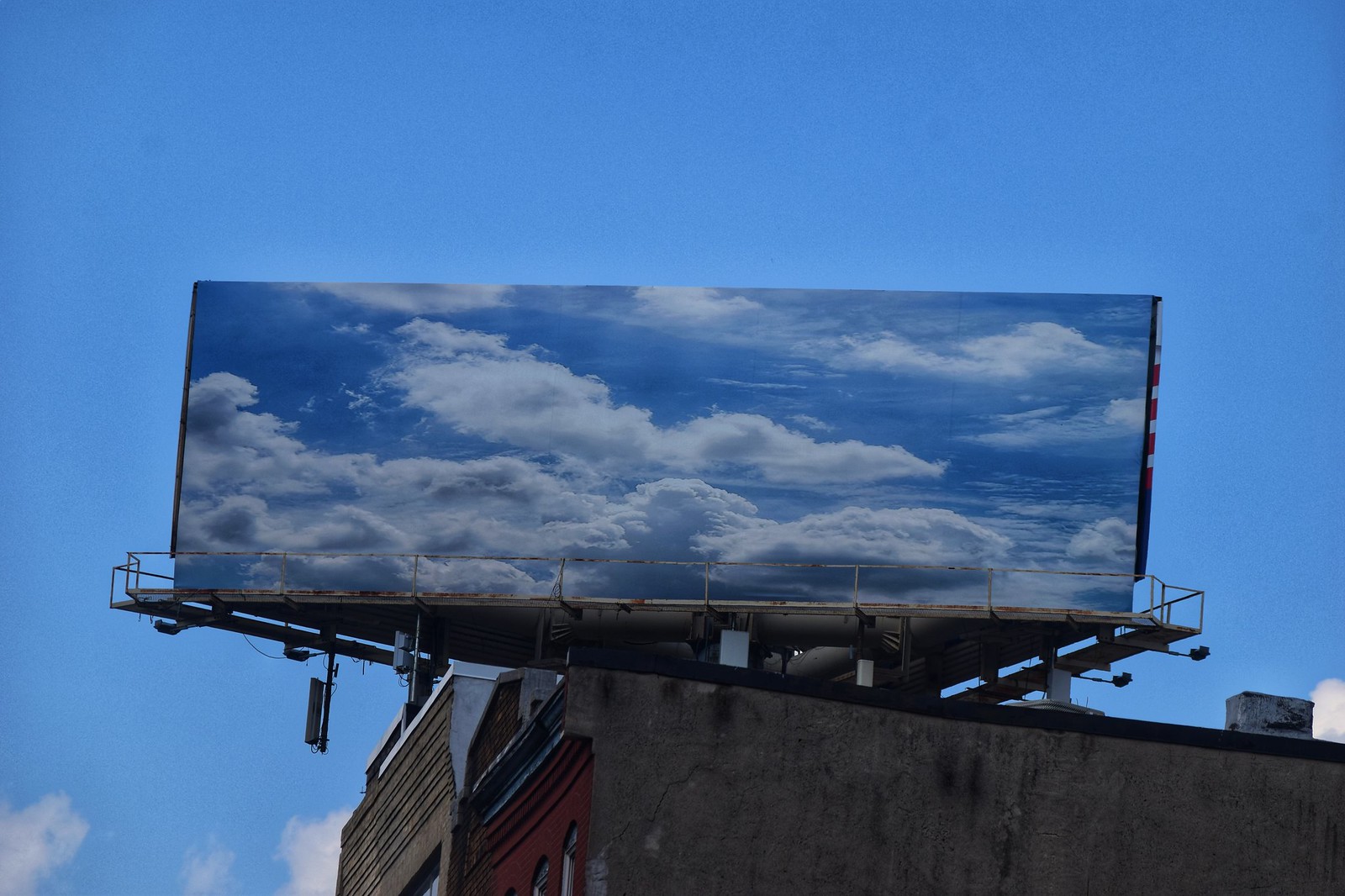This photograph captures a cityscape scene with a prominent billboard atop a multi-faceted building. The building itself features a striking combination of architectural elements: the side visible at the bottom exhibits a rugged gray concrete facade capped with a sleek black roof, while the front showcases a vibrant red wall punctuated by several windows. Adjacent to or possibly part of the same structure, another section reveals a modern aesthetic with smooth gray paneling. The background of the image is dominated by a serene, light sky blue expanse, accented with a smattering of white clouds near the lower portion. Dominating the upper skyline, the rectangular billboard displays an evocative image reminiscent of an aerial view through a plane window. This scene within a scene showcases a darker blue sky above a patchwork of voluminous, fluffy white clouds, resembling a vast, tranquil ocean below.